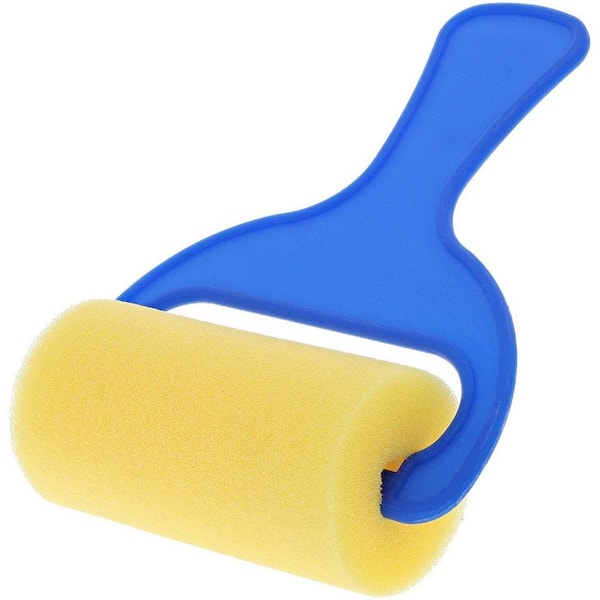This close-up image depicts a compact handheld tool on a white background, occupying approximately 90% of the frame. The tool features a distinctive blue plastic handle that splits into a Y shape. Between the two prongs of the Y, there is a light cream-colored foam roller with a hollow center, through which the handle is threaded and securely attached. The handle extends diagonally from the upper right-hand corner to the lower left-hand corner, emphasizing its ergonomic design suited for single-handed use. Although speculations vary, suggesting it might serve as a lint roller, a paint applicator, or a brush roller, the tool's small size and the foam material imply it is designed for detailed tasks rather than large projects.